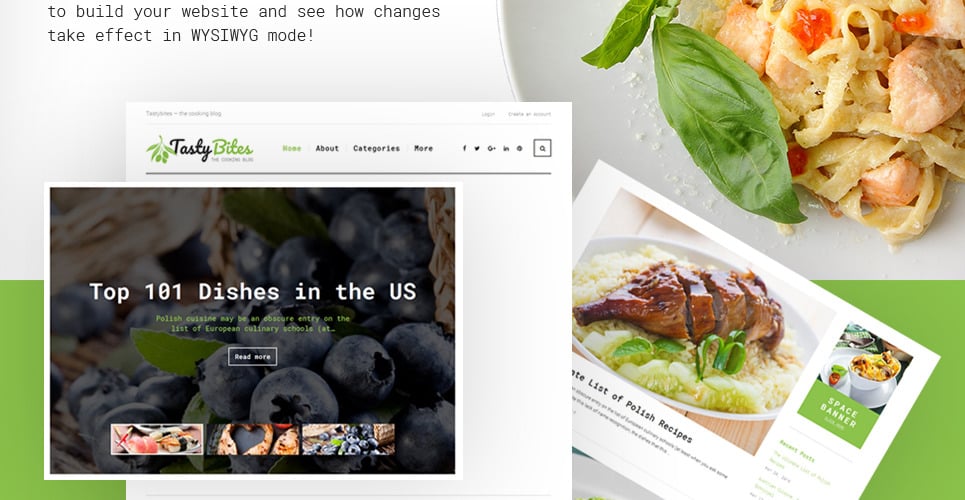This image depicts the front page of a food website called "Tasty Bites." Central to the page is a prominent white square, slightly positioned to the right, resembling a website within a banner. In the top-left corner, a black font message reads, "Build your website and see how changes take effect in WYSIWYG mode." WYSIWYG stands for "What You See Is What You Get," indicating direct visual feedback for web edits. Below, "Tasty Bites" serves as an example site for a website-building tool. The background of the banner features appetizing food imagery, with a dish prominently emerging from the top right side, emphasizing the culinary theme.